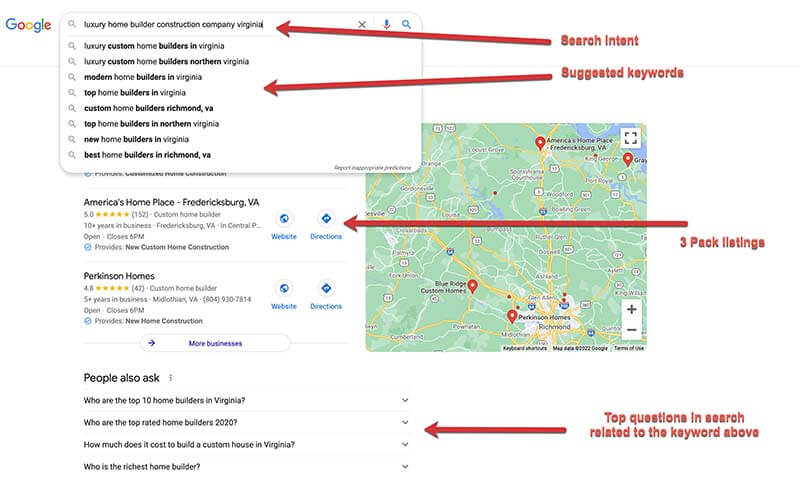The image depicts a Google search results page focused on the query “luxury home builder construction company in Virginia.” Prominently featured are several suggested keyword searches such as "luxury custom home builders in Virginia," "luxury custom home builders in Northern Virginia," "modern home builders in Virginia," "top home builders in Virginia," "custom home builders in Virginia," "top home builders in Northern Virginia," "new home builders in Virginia," and "best home builders in Richmond, Virginia." 

Additionally, a list of websites is displayed beneath these suggestions, including notable names such as America’s Home Place, based in Fredericksburg, Virginia, and Perkson Homes. The page also includes a section labeled "People also ask," featuring related questions like “Who are the top 10 home builders in Virginia?”, “What are the top-rated home builders in Virginia?”, “How much does it cost to build a custom house in Virginia?”, and “Who is the richest home builder in Virginia?”

A map is shown in the image, pinpointing the locations of some of these home builders, although one of the pictures is obscured by the overlay of the suggestions.